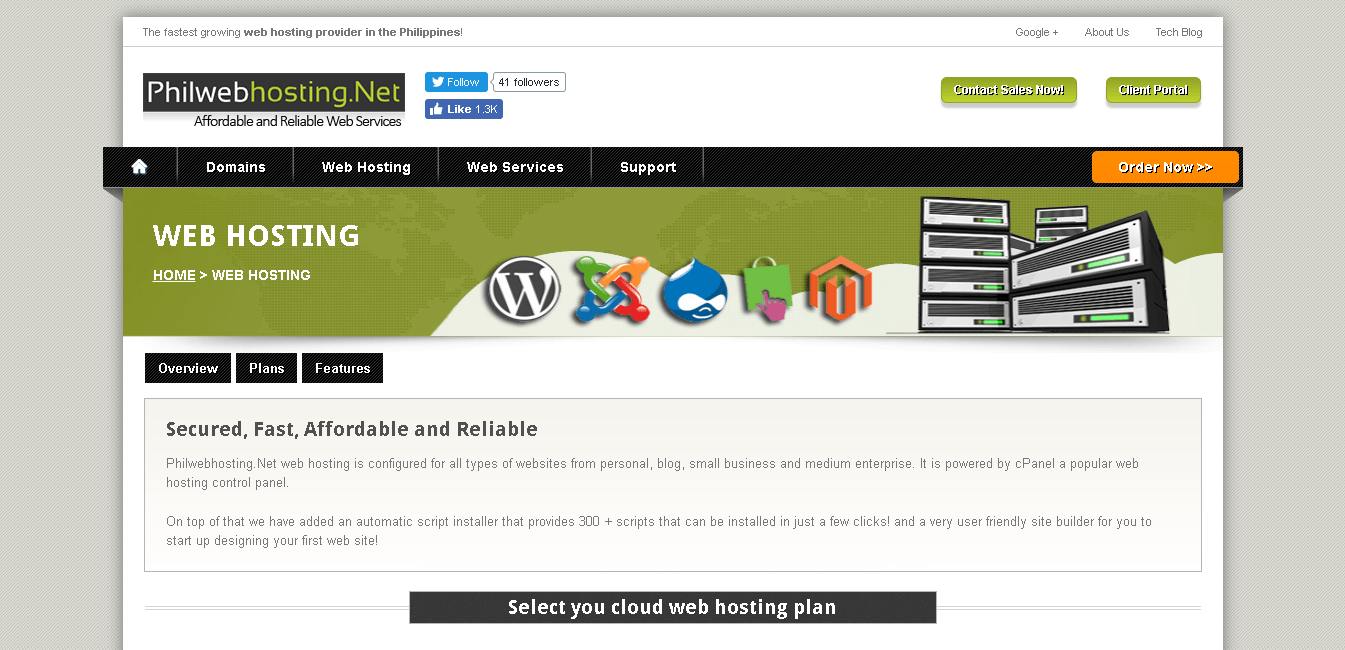The image depicts the homepage of a website called PhilWebHosting.net. The site's name features 'PhilWeb' in white text and 'Hosting.net' in green text. At the top, there's a white section that proclaims "Affordable and Reliable Web Services." This section includes interactive elements like a Twitter feed and a thumbs-up box to indicate likes, with several users having liked the site.

Below this header, there are two green boxes with white text that is unfortunately very blurred and difficult to read. The top section also contains some blue writing. Further down, the site organizes its services under categories such as "Domains," "Web Hosting," "Web Services Support," and highlights an "Order Now" button prominently displayed in an orange box on the right-hand side.

The main green section of the page provides more details about their web hosting services, labeled as "Home Web Hosting." This area features various computer icons in blue, green, orange, and black — the black icon has a "W" inscribed in it. To the right, there are several icons resembling computers or servers, depicted as black boxes with either silver or white fronts and green bars, numbering between six to eight units.

Below this icon section, the text reads "Overview," "Plans," and "Features," followed by keywords like "Fast," "Secured," "Affordable," and "Reliable." There is also a brief paragraph elaborating on these attributes, although it's challenging to read due to the poor legibility of the text.

Overall, the homepage aims to communicate the affordability, reliability, and various services offered by PhilWebHosting.net.